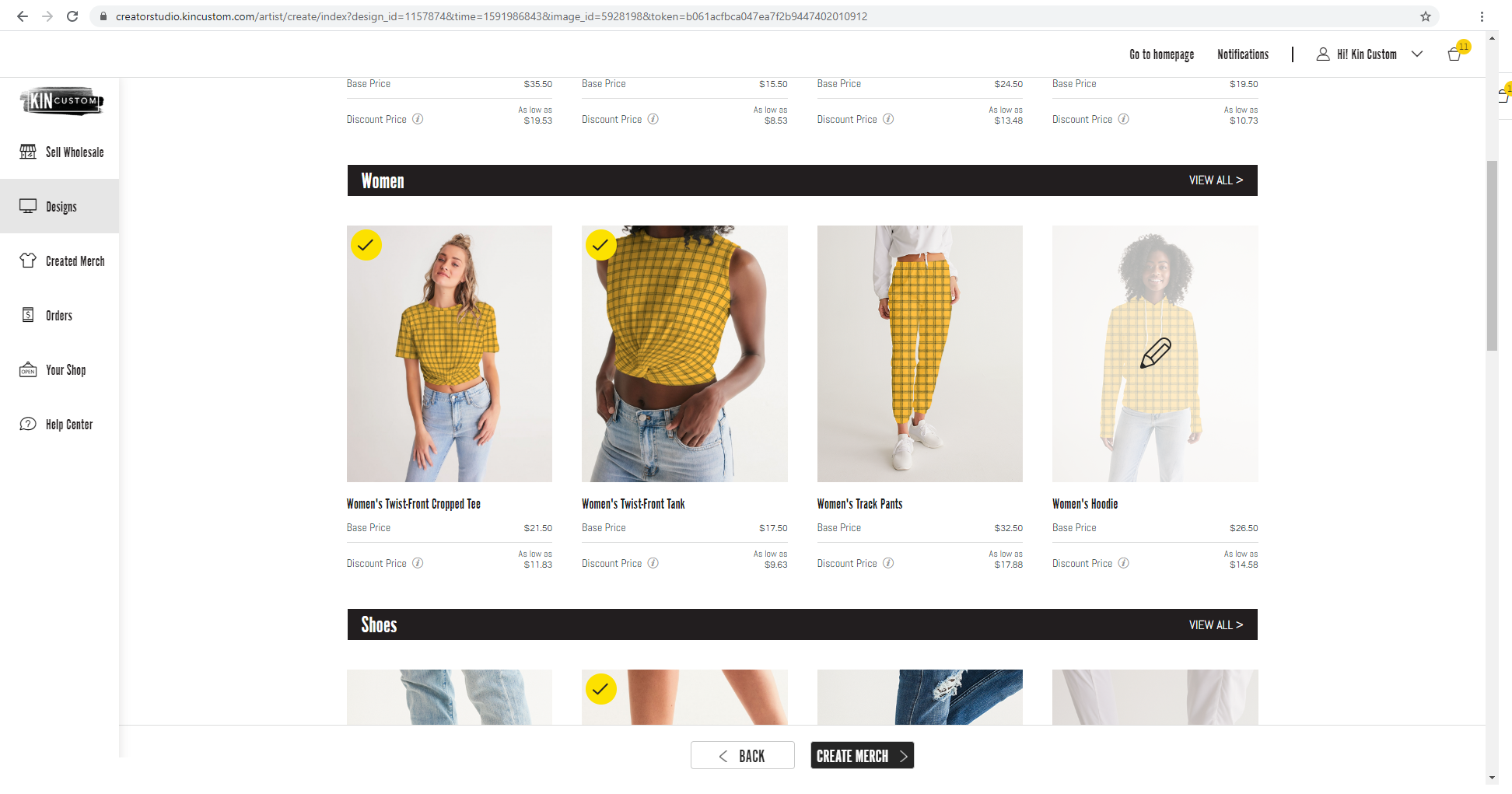Screenshot of Kint Custom's online store at creatorsstudio.kintcustom.com. The website features a variety of women's clothing and shoes prominently displayed in the center, including women's pants, twist front tanks, and hoodies, modeled by individual women. The interface has a clean, white background. The left sidebar offers navigational options such as: Sell Wholesale, Designs, Created Merch, Orders, Your Shop, and Help Center. At the bottom of the page, users have the ability to go back or create new merchandise. The top right corner includes links to the Homepage, View Notifications, and Account Management.